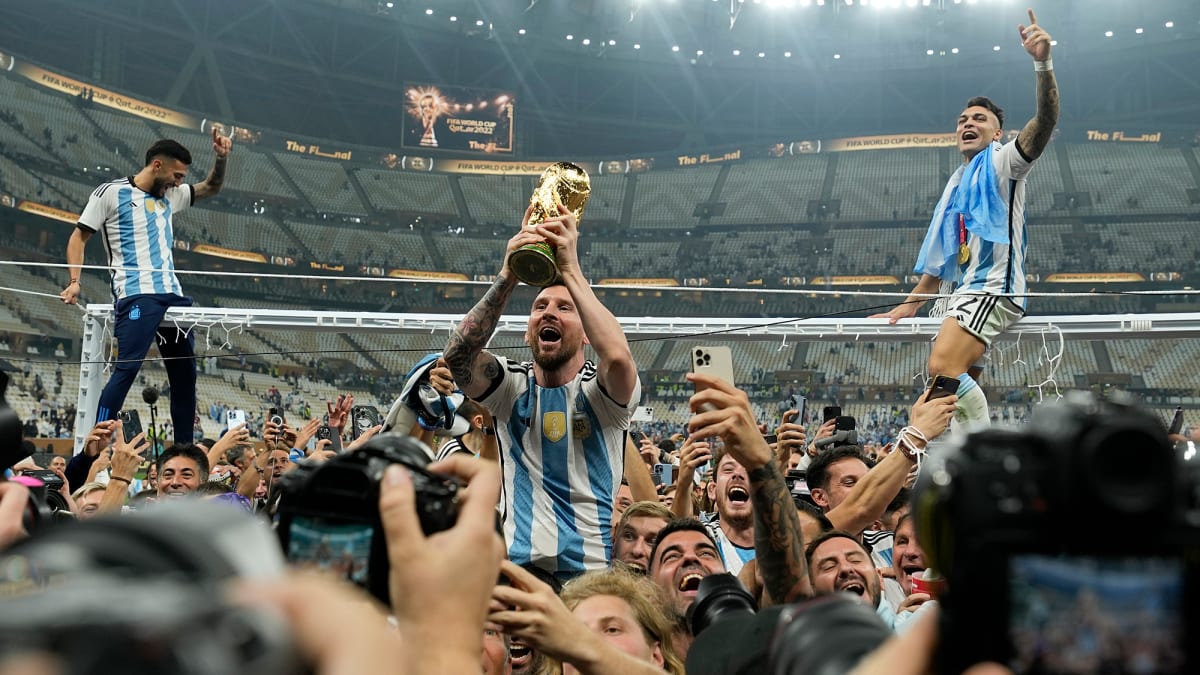The image captures the exhilarating celebration following Argentina's World Cup victory in soccer. At the forefront is Lionel Messi, the team's standout player, exuberantly holding a large gold trophy aloft. He wears a white jersey adorned with blue lines and a prominent gold shield at the center of his chest. His mouth is open in a joyful shout, and his tattooed arm is clearly visible. Flanking Messi are two teammates in similar jerseys; one to his right sports a blue scarf and is partially elevated, seemingly straddling the goal net, while the other to his left appears to be in mid-dance, also positioned atop the net. The backdrop reveals a massive stadium with dark gray, nearly black, seats sparsely occupied, and bright stadium lights towering above. The crowd surrounding the players is in high spirits, with faces beaming, hands raised, and the glow of smartphone screens capturing the moment. Photographers and reporters are visibly engaged in documenting this historic event, adding to the vibrant, joyous atmosphere of the scene.